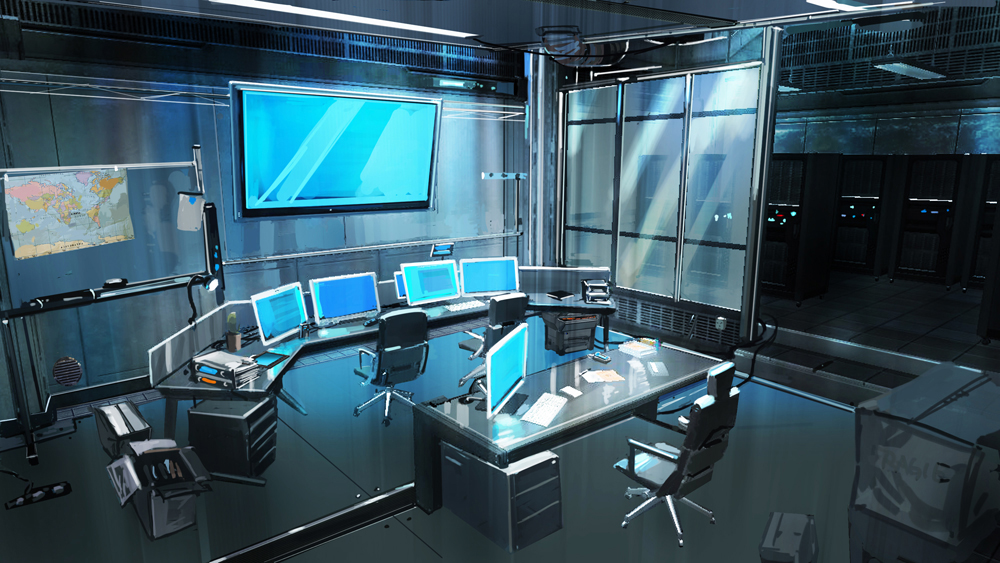This image depicts a digitally crafted illustration of a spacious, futuristic office environment. The room is characterized by its dark, glossy gray walls and floors that reflect light, giving it a sleek, modern look. Dominating the upper section of the space is a large, blue monitor, adding a splash of color to the otherwise monochromatic setting. In the background, there's a simple desk equipped with a chair, suggesting a secondary, more isolated workspace. In the foreground, a wide desk supports four blue monitors, reminiscent of a high-tech command center in a cartoon or a sci-fi movie. On the right side of the image, a black area with shiny white door panels hints at an adjoining room, possibly a dimly lit warehouse or storage area. The entire scene combines elements of sophistication and animation, creating a unique and engaging visual.